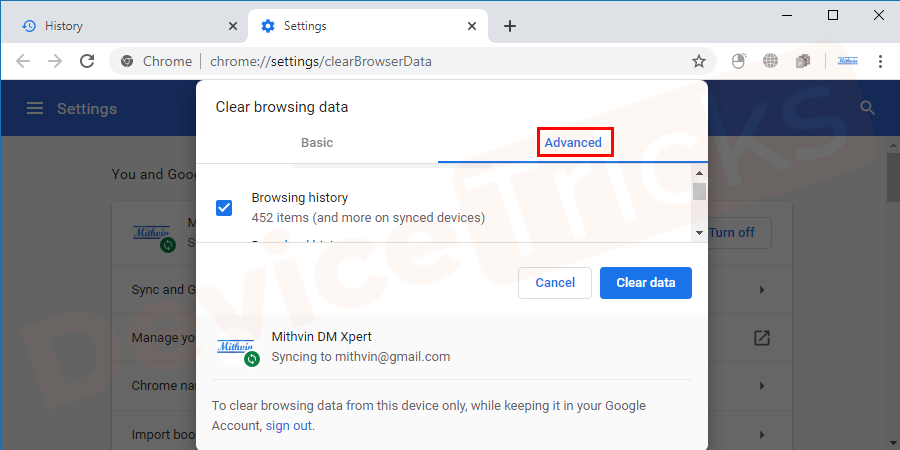The image is a detailed screenshot taken from a desktop or laptop displaying the Google Chrome browser in its "Settings" area. Chrome is set to light mode with a prominently bright and clean interface. The elements of the settings have a blue theme—checkboxes, buttons, and the header are all highlighted in blue, while the browser's background remains a light gray.

The screenshot focuses on the "Clear Browsing Data" section found at `chrome://settings/clearBrowserData`, specifically on the "Advanced" tab, which is distinguished by a red outline (added for emphasis). In this section, the user has selected the option to clear browsing data, with the checkbox for "Browsing history" being ticked and displaying 452 items ready to be cleared.

Below the list of checkboxes, two buttons are visible: a "Cancel" button and a blue "Clear data" button, both crucial for confirming or aborting the clearing process. Additionally, the bottom part of the screenshot reveals synchronization details, showing "Mythvin DM expert" syncing to the email address mythvin@gmail.com, indicating the account associated with the browser's data synchronization.

Overall, the image provides a comprehensive view of the user’s browser data clearing options, emphasizing their selection and offering a clear visual of the customizable settings in Chrome.